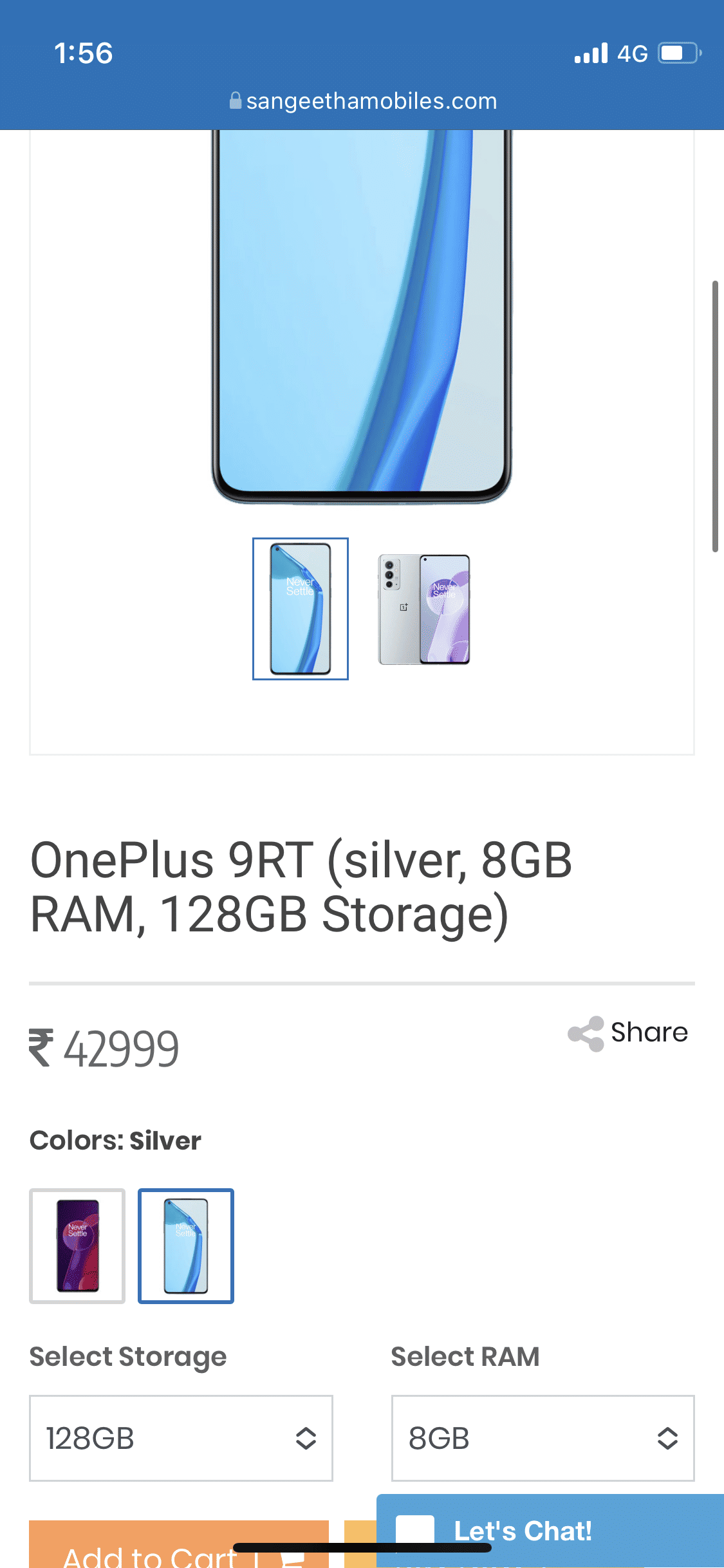This is a detailed caption for an image captured from a cell phone screen:

The photo is a screenshot presented in portrait orientation, consistent with the dimensions of a typical cell phone screen. On the top right corner, there is a thin, long gray scroll bar indicating that the page can be scrolled vertically. At the very top of the screen, a horizontal blue header spans across, displaying white text. On the top left, the time is shown as 1:56. In the center-bottom of the blue header, there's a link labeled "sayingethmobiles.com." To the top right, connectivity icons are visible, including a fully filled connection bar, a "4G" label, and a battery icon that is horizontally oriented with a white meter indicating battery life.

Below the blue header, the page background is white, displaying an image of a phone which is cut off at the top. The phone has a black frame and a blue background. Two highlighted images of the phone are displayed: one showing the full front view and the other showcasing the back. Below these images, black text reads "OnePlus 9RT, Silver, 8 GB RAM, 128 GB Storage." A border frames this description and below it, the price is listed as "$42,999" alongside a logo that is not identifiable, possibly indicating the currency.

Further down, there are options for selecting the phone color and storage capacity. The current selection is Silver, and there is an alternative selection with a purple and pink gradient-like color. Additional options allow adjustments for storage and RAM, with an "Add to Cart" button available for completing the purchase.